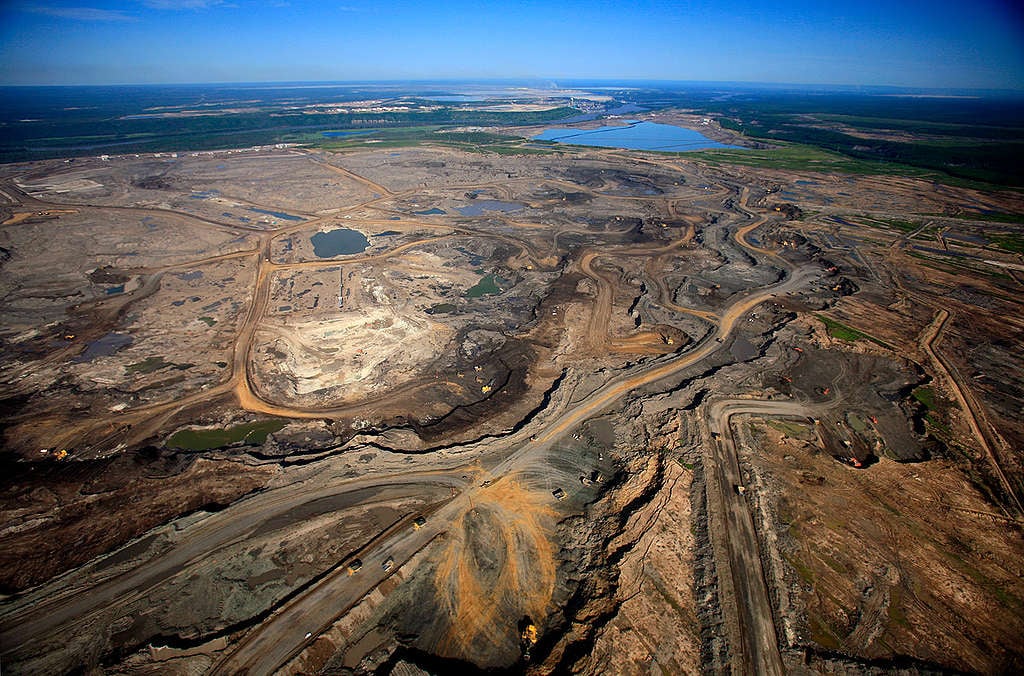This is a panoramic aerial daytime photo showcasing a massive, deforested and mined landscape that spans miles and acres. The image captures a labyrinth of dirt roads crisscrossing the terrain, facilitating the movement of various mining vehicles and tractors. The area predominantly consists of brown, black, and dirt-colored expanses with deep ditches and scattered pools of murky water, hinting at active resource extraction, possibly coal or other natural materials. Notably, the lower right corner of the photo displays a lot of black soil, resembling lava fields, with a road veering to the right and ending in more blackened earth. Flecks of orange suggestive of still-burning flames add a dramatic touch. Patches of green grass appear in the lower left and upper right corners, contrasting starkly against the barren landscape. In the background, a vast blue lake surrounded by green areas provides a striking juxtaposition to the desolate mined field, and beyond the lake, a white residential area suggests the presence of a nearby city. The clear blue sky completes the scene, highlighting the scale and scope of the mining operation.